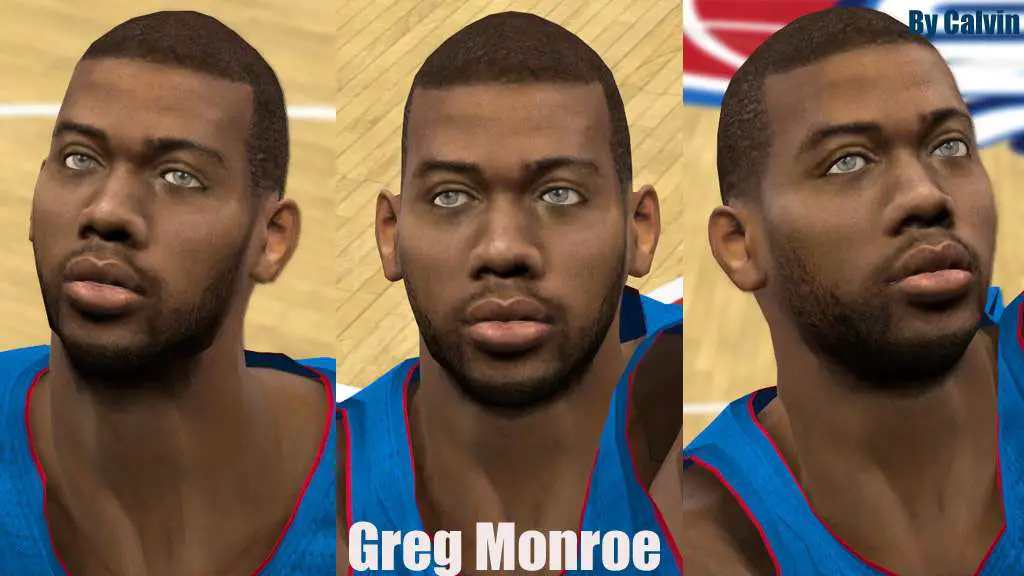This composite image features three side-by-side portraits of basketball player Greg Monroe on a basketball court. Each photo captures Monroe, a black athlete with short hair, blue or gray eyes, and a thin beard, mustache, and goatee, wearing a blue jersey with red trim along the sleeves and collar. 

In the leftmost picture, Monroe gazes to his left and slightly upward. The court beneath him is marked with prominent white lines. The middle image has Monroe looking directly into the camera, with his name, "Greg Monroe," displayed in white text at the bottom. The rightmost picture shows Monroe looking to his right and upward, revealing a court design featuring red, white, and blue elements behind him with the name "By Calvin" written beside his head. Monroe’s consistent appearance in all three images highlights his intense focus and athletic presence.